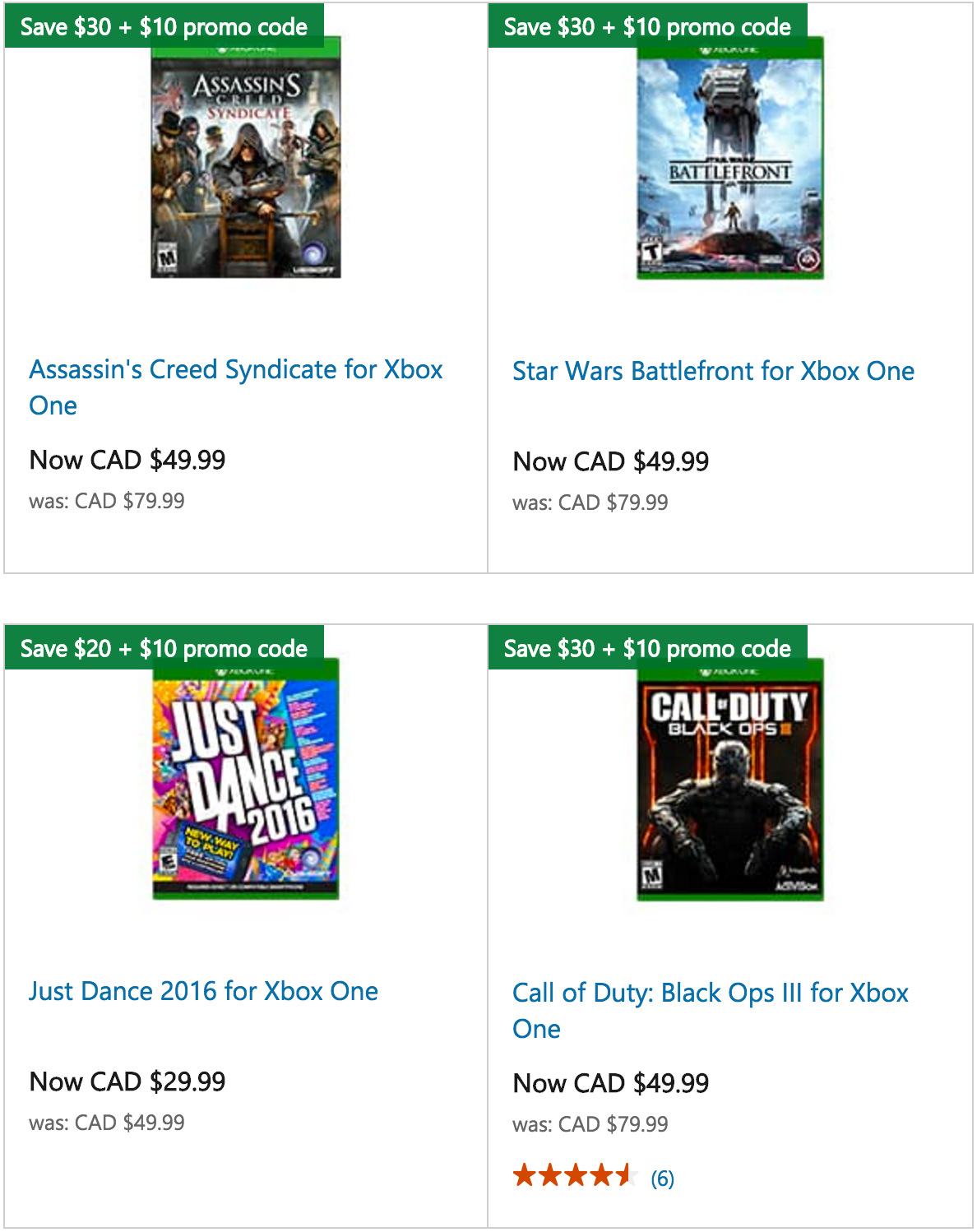The image displays a selection of video games available for Xbox One, highlighted with promotional savings. At the top, a green tag announces a $30 discount along with a $10 promo code. 

1. **Assassin's Creed Syndicate**: Priced at CAD $49.99 (originally CAD $79.99), the cover features several characters, with the main character prominently seated in a chair, all dressed in old-fashioned attire.
   
2. **Star Wars Battlefront**: Also available for CAD $49.99, down from CAD $79.99, though no additional description about the cover is provided, we can assume typical Star Wars themed artwork.

3. **Just Dance 2016**: Priced at CAD $29.99, discounted from CAD $49.99, and tagged with "Save $20 plus $10 promo code", the cover likely features energetic dance-related imagery, characteristic of the series.

4. **Call of Duty: Black Ops 3**: Priced at CAD $49.99, originally CAD $79.99, the cover showcases a character wearing a mask and armor against a backdrop of yellow and red hues. The game has a 4.5-star rating based on 6 reviews. 

All pages are presented with a white background, the video game covers, and blue text, emphasizing the promotional details.